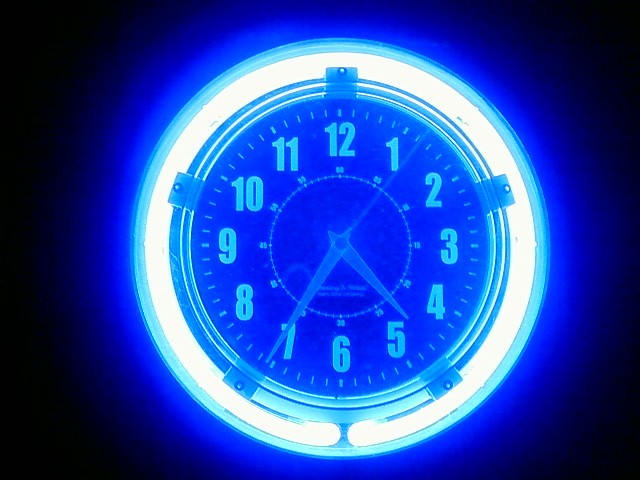This image showcases a striking wall clock set against what seems to be a black wall or shadowed background. The clock's outer rim is adorned with a vibrant, neon-blue light that forms a luminous circle, casting a range of blue hues onto the surrounding area. At the heart of the clock, stark white numbers stand out against a dark, possibly black base. The clock's hands exhibit a translucent quality, adding a modern touch to its design. Additionally, there is an inner circle within the clock, also marked with numbers in increments of five, accompanied by minute indicators along the edge to denote the seconds. Overall, the clock's vivid blue illumination and contrasting elements create a visually captivating and modern timepiece.